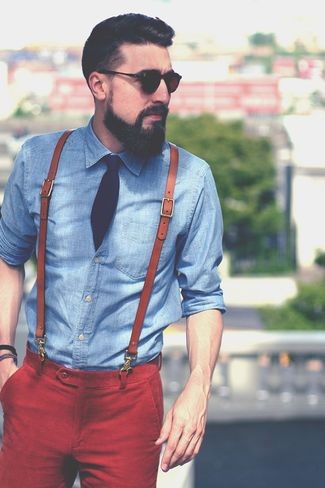The photo captures a middle-aged white man with very dark, close-cropped hair, posing outdoors in front of a blurry backdrop suggestive of buildings and trees, possibly on a balcony or rooftop. He sports dark sunglasses and a neatly manicured black beard. Dressed in a light blue linen button-up shirt with the sleeves rolled up to his elbows, the man also wears a matching blue tie tucked into his shirt. His bright red jeans are secured with leather suspenders of the same vibrant hue. His right hand rests casually in a pocket, showing either a watch or bracelets on his wrist. The overall focus is on his stylish appearance while he gazes off to the side.